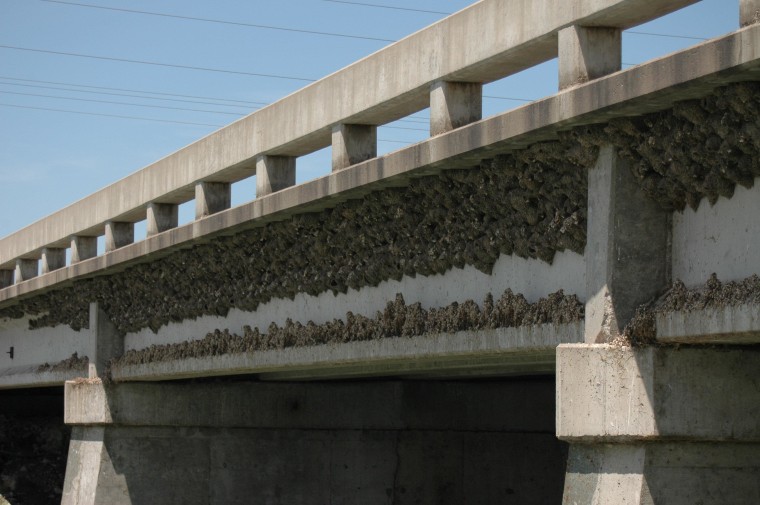The image is a detailed side view of a heavy concrete bridge on a bright, sunny day with a clear blue sky and no clouds. Perpendicular to the bridge, several power lines stretch across the background. The bridge, primarily composed of weathered gray concrete, features a railing along its upper edge. This railing, supported by regular-sized rectangular supports, is prominently discolored and dirty.

The underside of the bridge is particularly dark and heavily encrusted with brownish-gray lumps, which may be insect nests, possibly wasp or dirt dauber nests, or some form of animal pods or growth such as moss or lichens. These structures are thickly clustered along the upper and lower edges of the bridge, creating a textured and somewhat grimy appearance. The primary focus of the photograph is these growths or nests that darken and mar the surface of the concrete. 

Below the bridge, large concrete supports hint that it spans over water or another road, but this aspect remains unclear. The overall color palette of the image is dominated by various shades of gray and white, juxtaposed against the blue sky and black electrical wires.